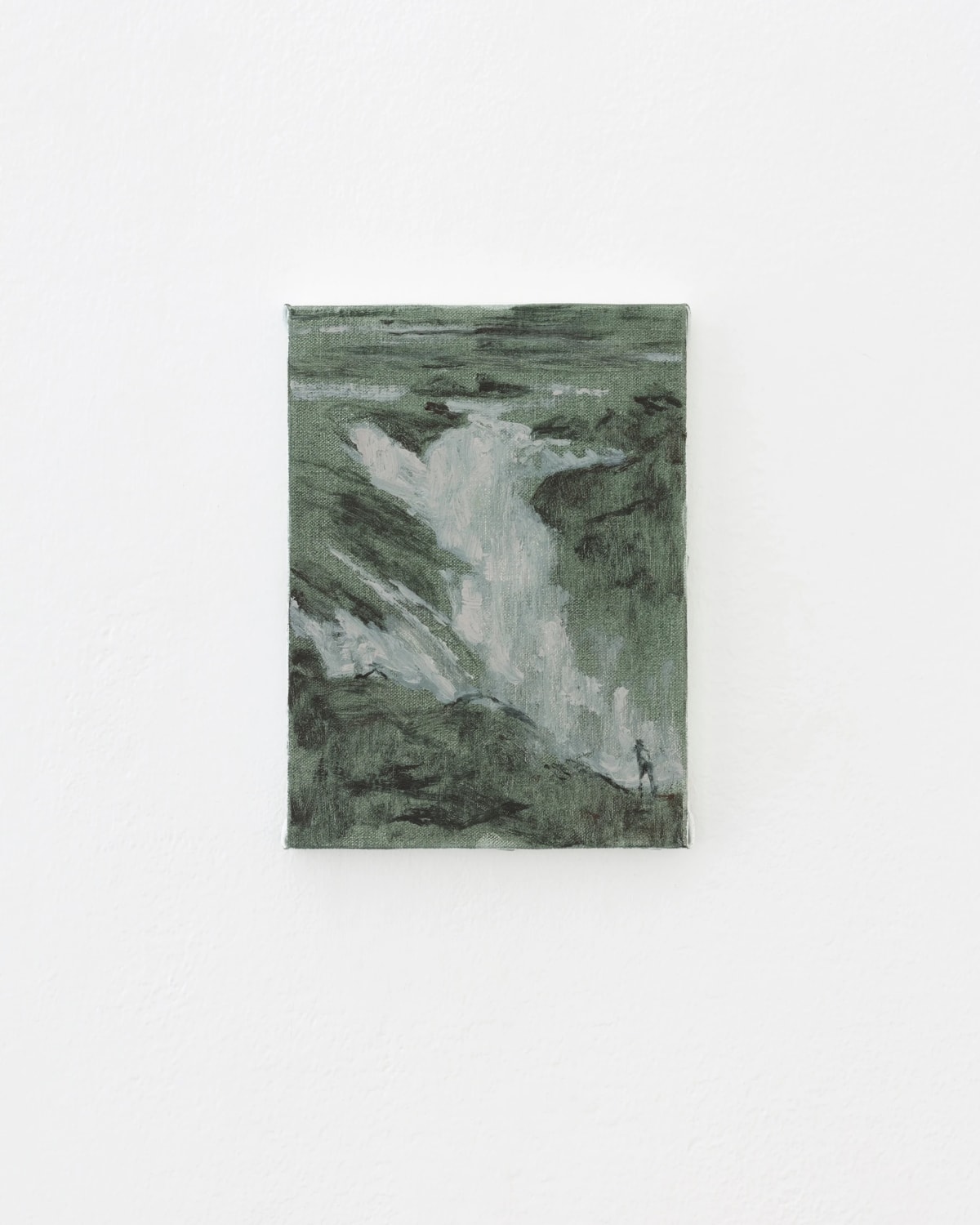The image in question is a minimalistic painting centered on a canvas with a plain gray background framed in white. The painting primarily employs monochrome shades of green, gray, and black, with a striking white element depicting a waterfall cascading down the center. The style is very abstract and loose, creating an open field for interpretation; what appears to be a waterfall to some might be interpreted as an iceberg or glacier by others. In the bottom right-hand corner, there is a small figure, likely a person, possibly a photographer or hiker, standing on what seems to be a cliff or rocky edge, facing the waterfall. The figure is minimally detailed, adding to the painting’s simplicity and ambiguity. The surrounding landscape includes hints of a forest and rocky terrain, enhancing the natural, serene, yet enigmatic ambiance of the scene.